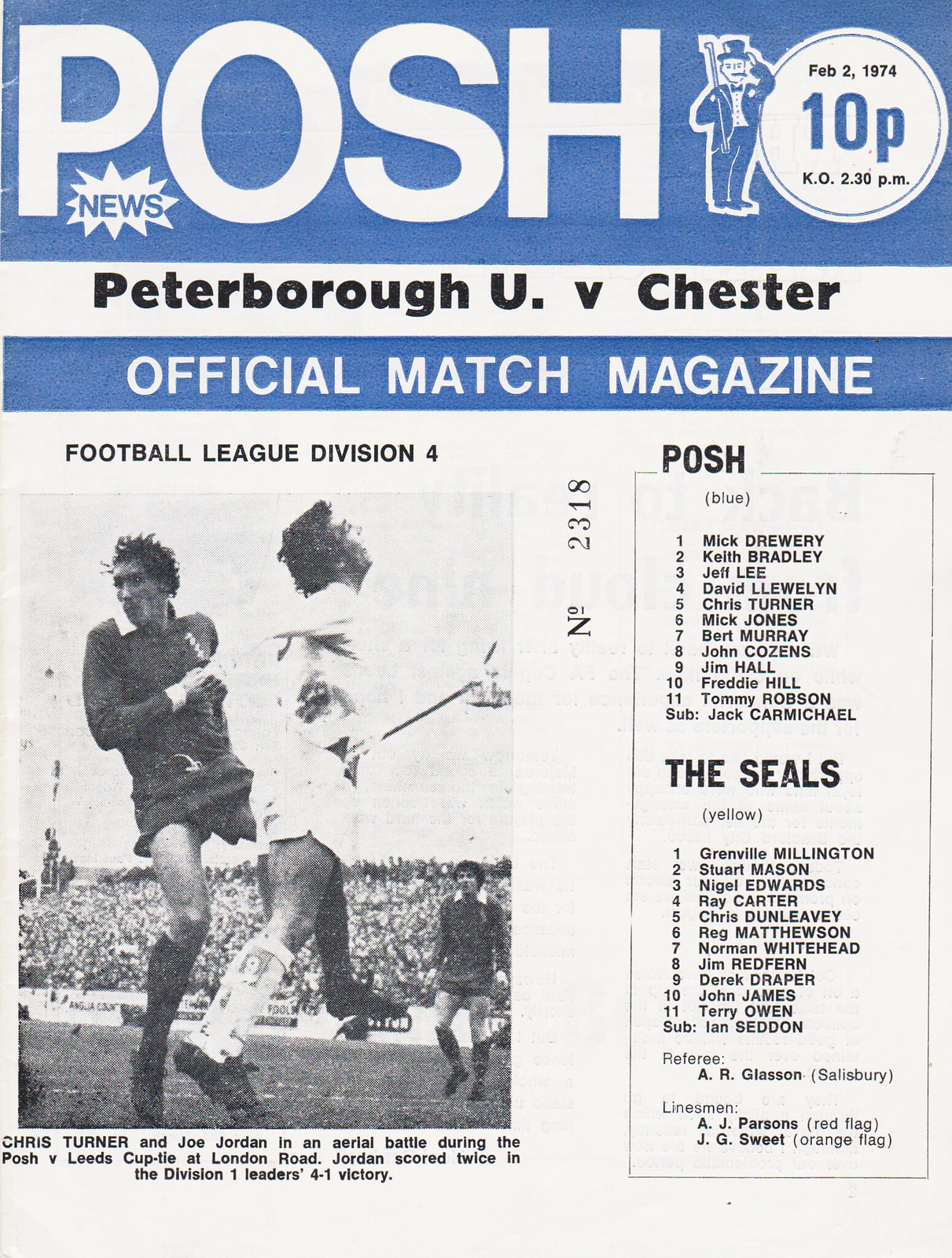This image depicts a vintage front page of a magazine titled "Posh News" dated February 2, 1974, priced at 10 pence. Dominating the cover is a stylish illustration of a golfer dressed in a suit, bow tie, and hat. Below the title, the magazine details a football match between Peterborough United and Chester, labeled as an "official match magazine" for the Football League Division Four. 

There is a prominent black-and-white photograph centered on the cover, showing two football players leaping into the air during a match. One player is dressed in a dark uniform while the other is in a light one, with a crowded arena visible in the background. The text above the photo reads "Football League Division Four," confirming that it is indeed a soccer match scene. Moreover, the left player appears to be Jim Jordan, who notably scored twice in the pictured match between Posh and Chester.

On the right side of the cover, both teams' rosters—Posh and Seals—are listed, providing a detailed breakdown of the players involved in this historic match.